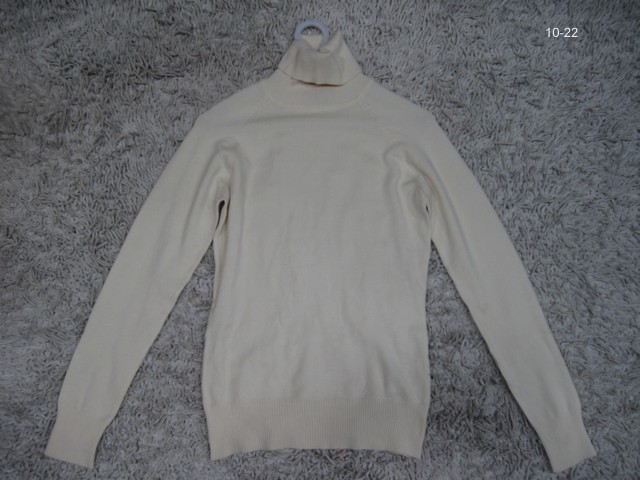In the dimly lit image, a plain white or cream-colored turtleneck sweater is displayed on a soft, gray shag carpet. The turtleneck, with its collar folded over, and long sleeves slightly angled downwards at about 30 degrees, is arranged on a white plastic hanger. The sleeves and bottom of the sweater feature ribbed cuffs, and there are a few slight wrinkles suggesting it wasn't laid completely flat. The soft, curly textures of the plush gray carpet underneath create a cozy background. In the upper right corner of the image, the numbers "10-22" are superimposed, possibly indicating the date the photograph was taken. The lighting is even, although slightly darker towards the bottom, creating gentle shadows and highlights that emphasize the sweater's texture and the plush appearance of the carpet.